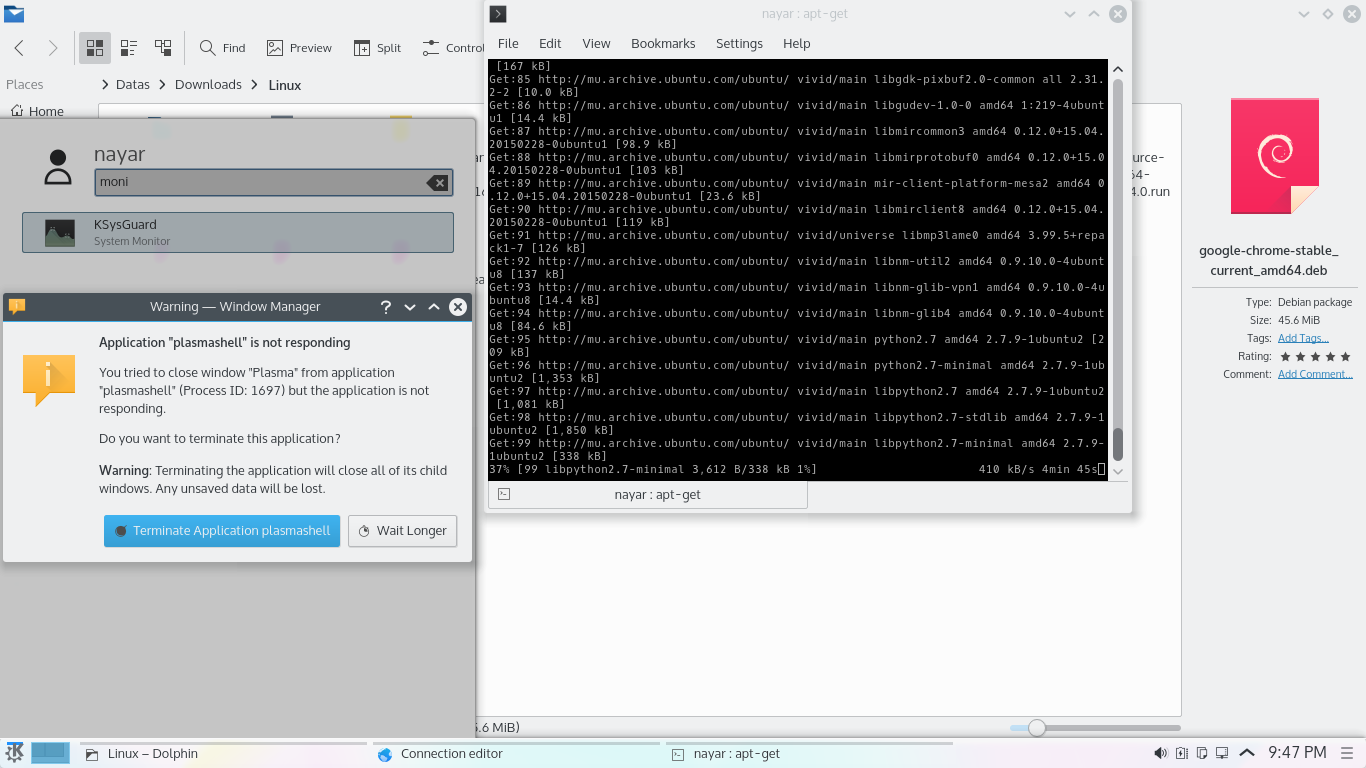The image depicts multiple overlapping windows on a computer screen. The foreground features a dark-themed coding interface, densely populated with white text indicative of programming or script editing. The top of this window reveals a traditional menu bar with tabs labeled "File," "Edit," "View," "Bookmarks," "Settings," and "Help." 

Behind this primary window, a side window presents a personal profile titled "Nayar," which is accompanied by a warning message from the window manager, stating "Application plasmatical is not responding." Adding to the clutter, a third window positioned at the back appears to display a white document with partial text, though the specifics are obscured by the foreground windows.

On the right side of the screen, there is a sidebar labeled with terms like "Google Chrome," "staple," "current," followed by additional unclear information. The bottom of the screen mimics a typical computer interface, featuring various tabs and widgets, completing the representation of a multitasking digital workspace.